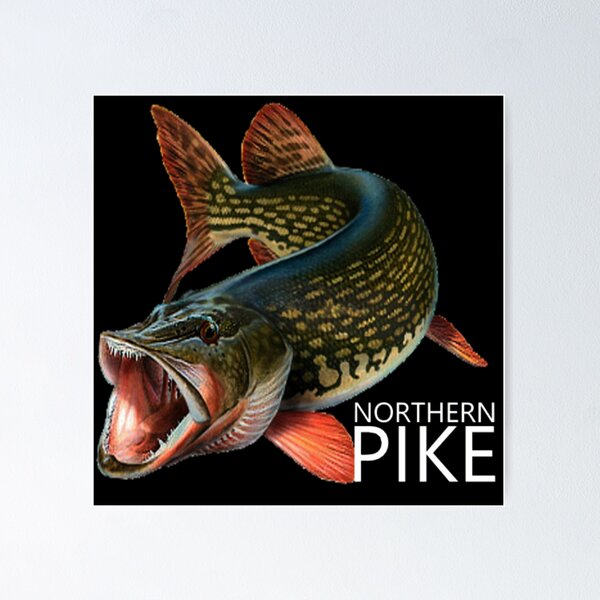The image is a vividly detailed product photograph of a square-shaped poster set against a neutral, solid grey background. The poster itself features a thin white border along all its edges. Dominating the poster is a striking image of a Northern Pike, set against a solid black background. The fish is depicted with its head facing forward, its mouth wide open, revealing sharp white teeth. The Northern Pike is distinguished by its green back adorned with light green spots, a white stomach, and vibrant red fins and tail fins that are speckled with green and brown spots. In the bottom right corner of the poster, the words "Northern Pike" are elegantly printed in white, with "Northern" placed directly above "Pike," the latter appearing in a larger font. The clarity of the image is exceptionally high, highlighting the intricate details and colors of the fish against the contrasting black background. The overall presentation of the product is clear and well-lit, making it visually appealing.